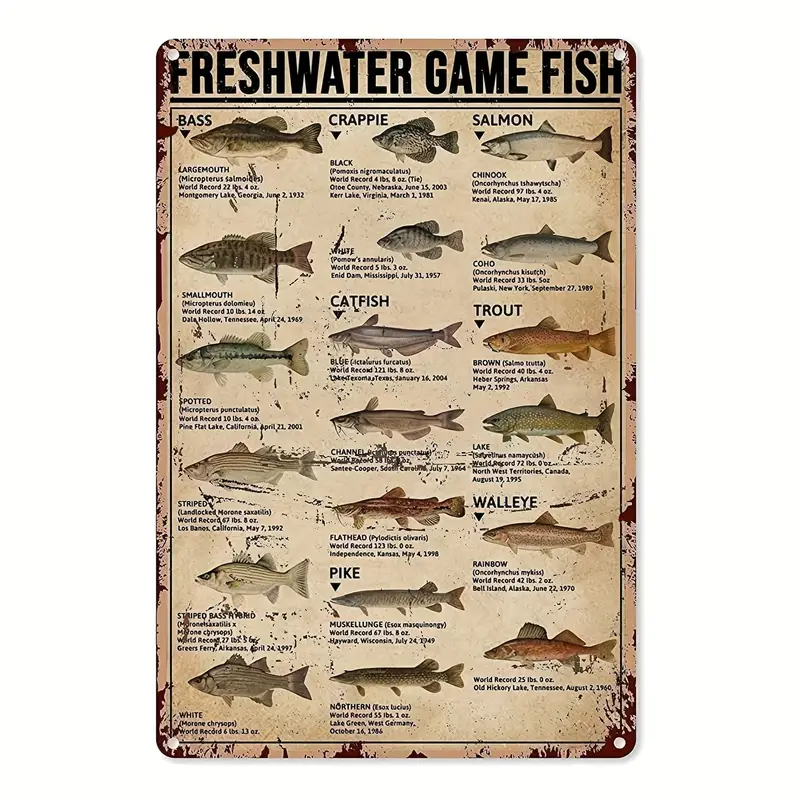The image titled "FRESHWATER GAME FISH" is a worn vintage metal sheet, illustrated in a tall rectangular format with holes in all four corners for mounting. The sign, which appears to have been in use for a long time, shows signs of wear including nicks and worn edges with red smatterings around it. The background is beige, and there are three rows of intricately drawn freshwater game fish, each with labels detailing the specific types. The fish categories include bass, crappie, catfish, pike, salmon, trout, and walleye. Within each category, the labeled subtypes are: 

- Bass: largemouth, smallmouth, spotted, striped, striped bass hybrid, and white.
- Crappie: black and white.
- Catfish: blue, channel, and flathead.
- Pike: muskellunge and northern.
- Salmon: chinook and coho.
- Trout: brown and lake.
- Walleye: rainbow.

Beneath each illustration, there are brief descriptions and Latin names of the fish. The weathered sign also features an old record detail at the bottom, noting a world record walleye weighing 25 pounds, caught at Old Hickory Lake, Tennessee, on August 2, 1960. The sign is encompassed by a black border, giving the vintage artwork a framed appearance, which adds a classic touch to this informative depiction of freshwater game fish.